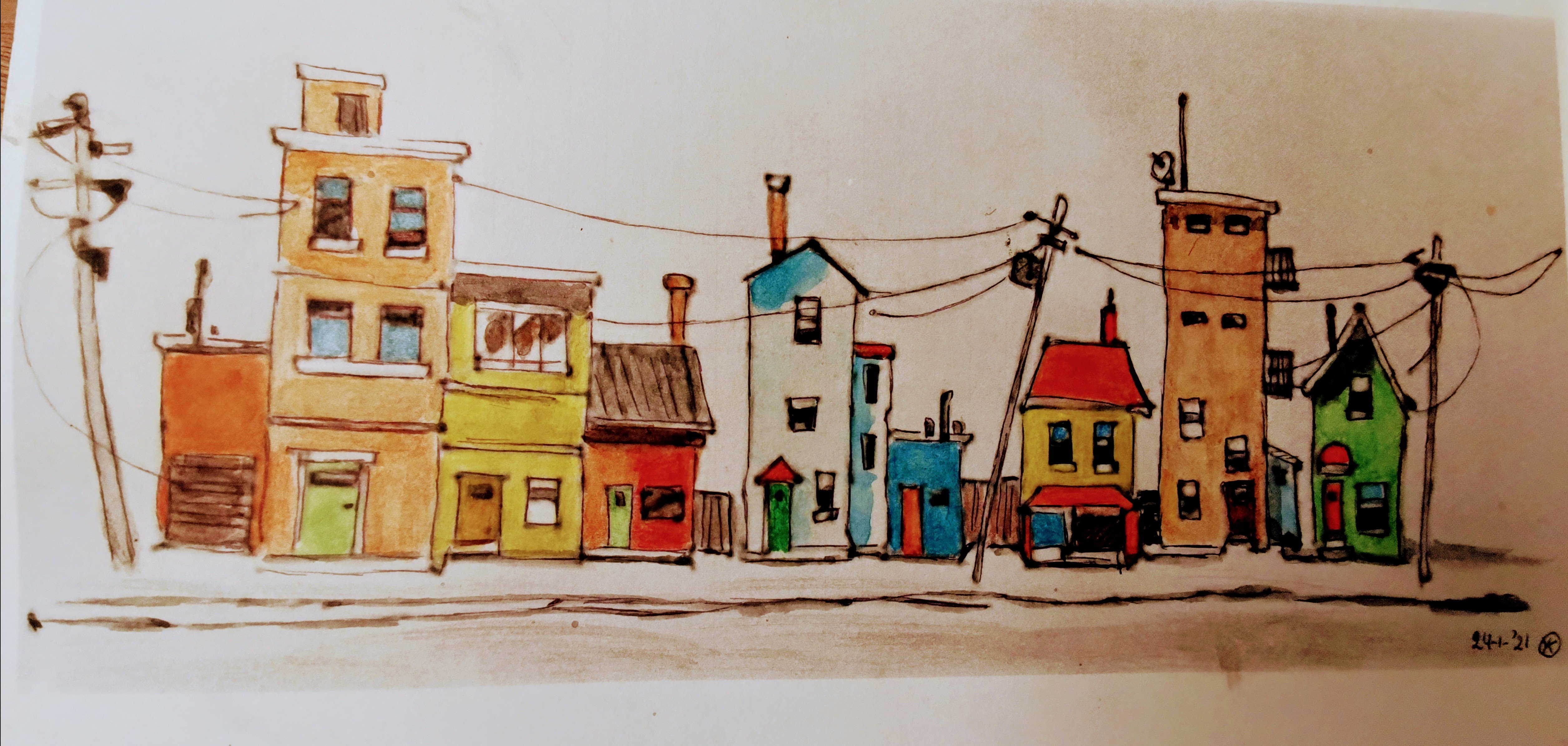This image is a photograph of a hand-drawn illustration on a piece of paper, likely placed on a table. The upper left corner hints at the table surface beneath the paper. The drawing captures a small segment of an urban street from the artist's perspective. Notably, the scene only depicts one side of the street, showing no opposing buildings. 

The street is lined with a series of tightly packed buildings, reminiscent of a bustling cityscape such as New York City, where space is at a premium. The buildings vary in height, with many being at least two stories tall, and a few rising to three stories. Each building has its own unique color, contributing to a vibrant yet congested atmosphere. A couple of the structures appear abandoned, their windows and doors boarded up. Overhead, power lines crisscross the scene, adding to the urban feel. 

The foreground includes details of the sidewalk and a portion of the street, grounding the setting in a recognizable city environment. The artist's signature and a copyright symbol are neatly placed in the bottom right corner of the paper, affirming the originality of the artwork.